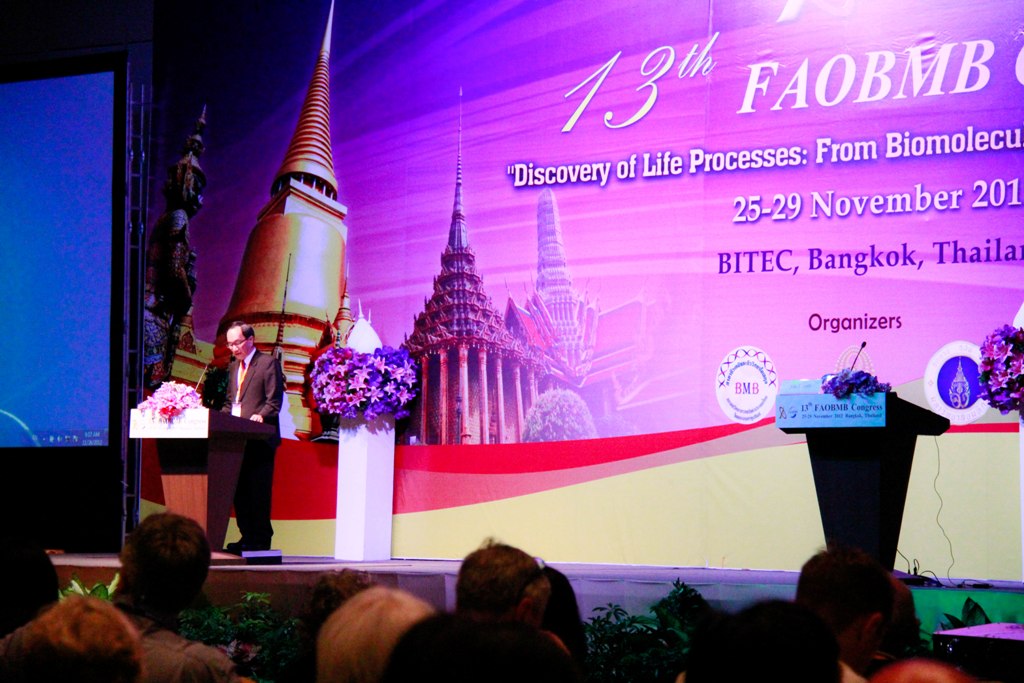An older Asian gentleman, dressed in a black suit and white shirt, is speaking on a decorated stage at a conference in Bangkok, Thailand. The event, identified as the 13th FAO BMB, focuses on the discovery of life processes from biomolecular studies and takes place from November 25th to 29th, though the specific year is cropped out from the image. The stage features a richly decorated podium adorned with various flowers, and a vibrant, colorful poster forms the backdrop. In the audience, one can see heads with various hairstyles. To the right of the speaker, there is an additional podium that remains unoccupied. A prominent tower or religious temple, evocative of Thailand's architecture, is visible in the background, reinforcing the location of the event.